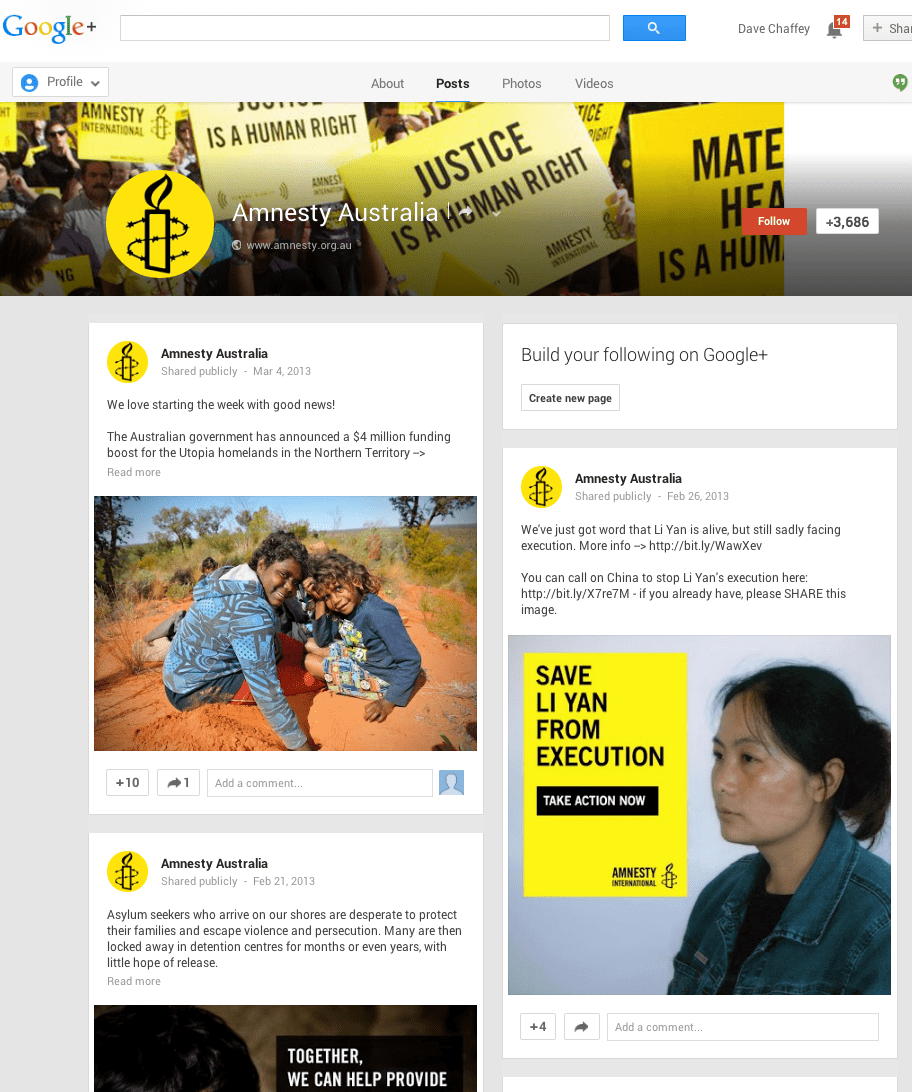The image is a screenshot of a Google+ page belonging to "Amnesty Australia," a social networking profile similar to Facebook. In the upper left-hand corner, the Google+ logo is visible, indicating the platform. The profile picture of Amnesty Australia features a yellow background with a black lit candle encircled by a backward "S."

Several posts are visible on the page, each detailing various human rights issues. One post celebrates a positive development: "We love starting the week with good news. The Australian government has announced a four million dollar funding boost for the Utopia homelands in the Northern Territory." Another post updates on a critical situation: "We've just got word that Leon is alive but still sadly facing execution. More info [link]. You can call on China to stop Leon's execution here [link]. If you already have, please share this image." Lastly, a post highlights the dire circumstances faced by asylum seekers: "Asylum seekers who arrive on our shores are desperate to protect their families and escape violence and persecution. Many are then locked away in detention centers for months or even years with little hope of release."

This detailed snapshot provides a glimpse into Amnesty Australia's advocacy work and the pressing human rights issues they are addressing.